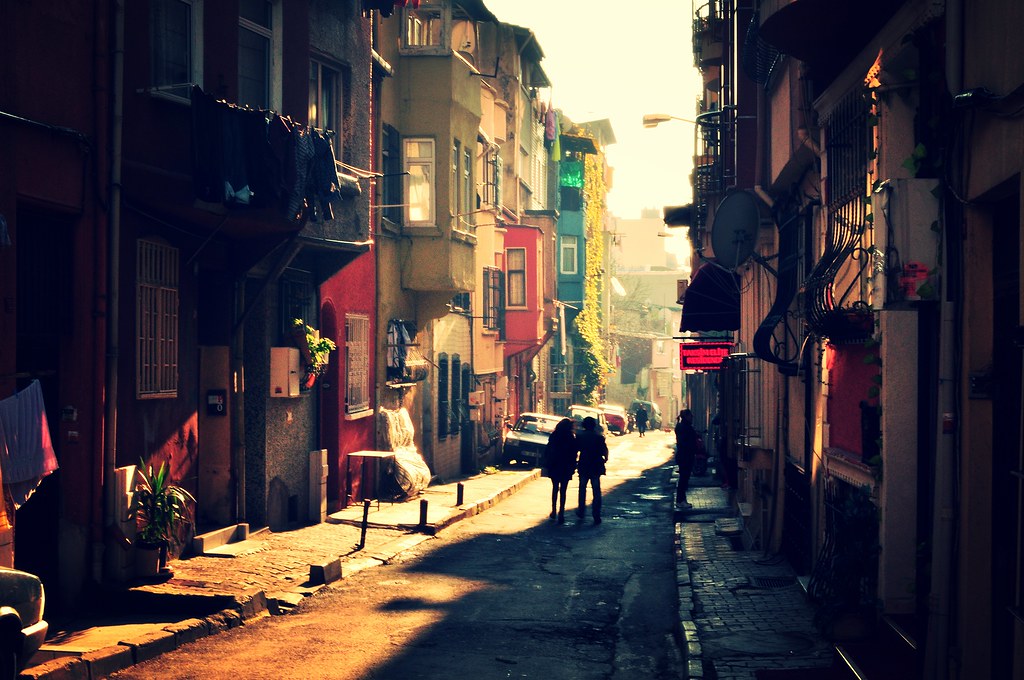The image is a highly artistic, high-contrast depiction that looks like it could be found on deviantART, possibly rendered or expertly photographed. It captures a vibrant, possibly European street scene at sunset, between two rows of colorful, three-story high houses. The sun casts a striking beam of light through the roadway, leaving the rest of the street in dramatic shadows. The buildings are painted in rich hues of red, light olive, deep green, and orange, each displaying unique elements like bay windows, balconies with flowers, and hanging clothes. Two silhouetted figures, possibly females, walk away from the camera down the cobblestone or brick street, which shows signs of wear and decay. Parked cars are tucked to the sides, and other notable elements include a satellite dish, barred windows, a street light, and a red business sign, all contributing to an old-world charm reminiscent of San Francisco or a South American city.